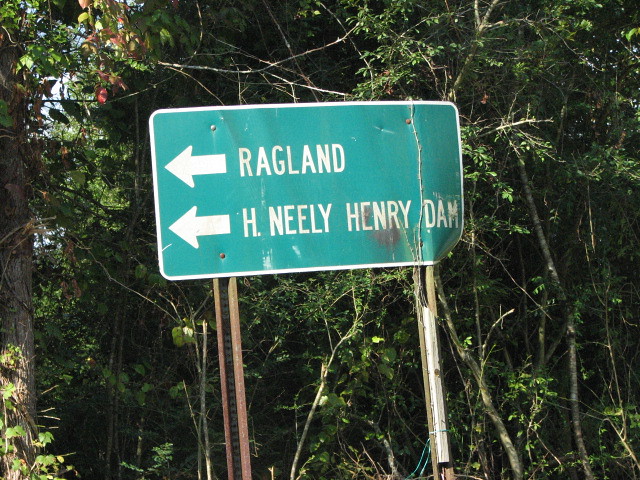In this photograph, there is a notably old and weathered road sign, positioned on the side of the road amidst dense forest vegetation. The sign, which has a rectangular shape and displays a bluish-green hue due to years of fading, is supported by two worn posts - one on the right that has a white tint with brown reinforcement and another on the left that is brown and rusting. The sign itself, which points left, has two arrows both aiming in that direction. The top arrow directs towards "Ragland" while the bottom arrow indicates the way to "H. Neely Henry Dam," although the word "Dam" appears creased as if the sign has been bent. Surrounding the old sign are trees with trunks of varying thickness in shades of gray and brown. Their branches are adorned with green leaves, predominantly dark green with some lighter shades, and a few exhibiting a reddish hue. Vine-like vegetation is beginning to encroach upon the sign, adding to its worn and almost consumed appearance.